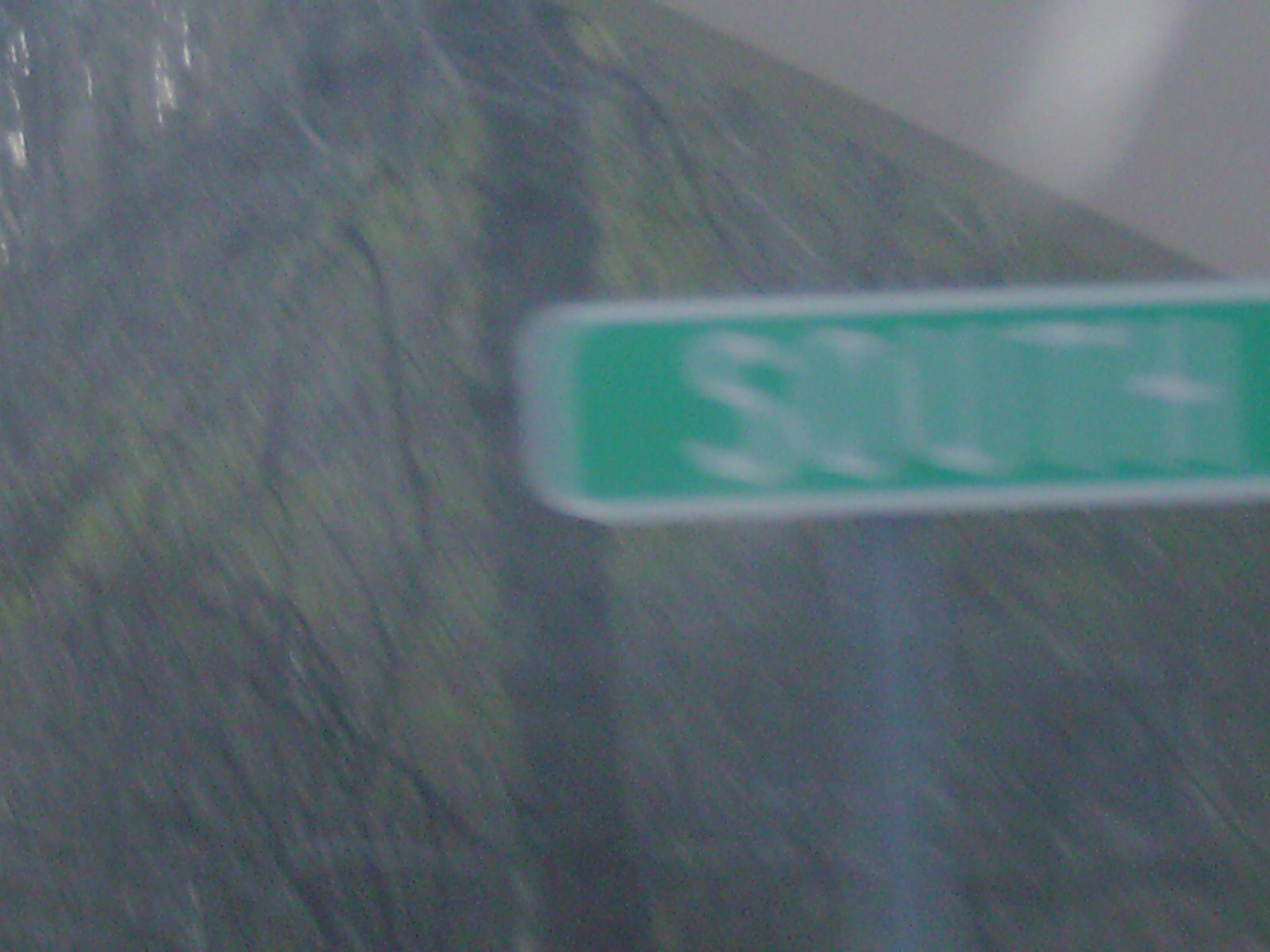The image is a slightly horizontally rectangular frame characterized by excessive blurriness. The background features what appears to be a dark tree, almost black in color, with slender branches interspersed with patches of green foliage. In the lower right corner of the frame, there's a very fuzzy, heavily blurred silver pole that extends upward from the bottom right. At the top of this pole is a green traffic sign with a white border, reminiscent of a standard road sign. However, the right side of the sign is cut off by the edge of the frame, so only the word "SOUTH" in white letters is visible. The overall effect is a somewhat abstract and impressionistic scene due to the significant blurring.